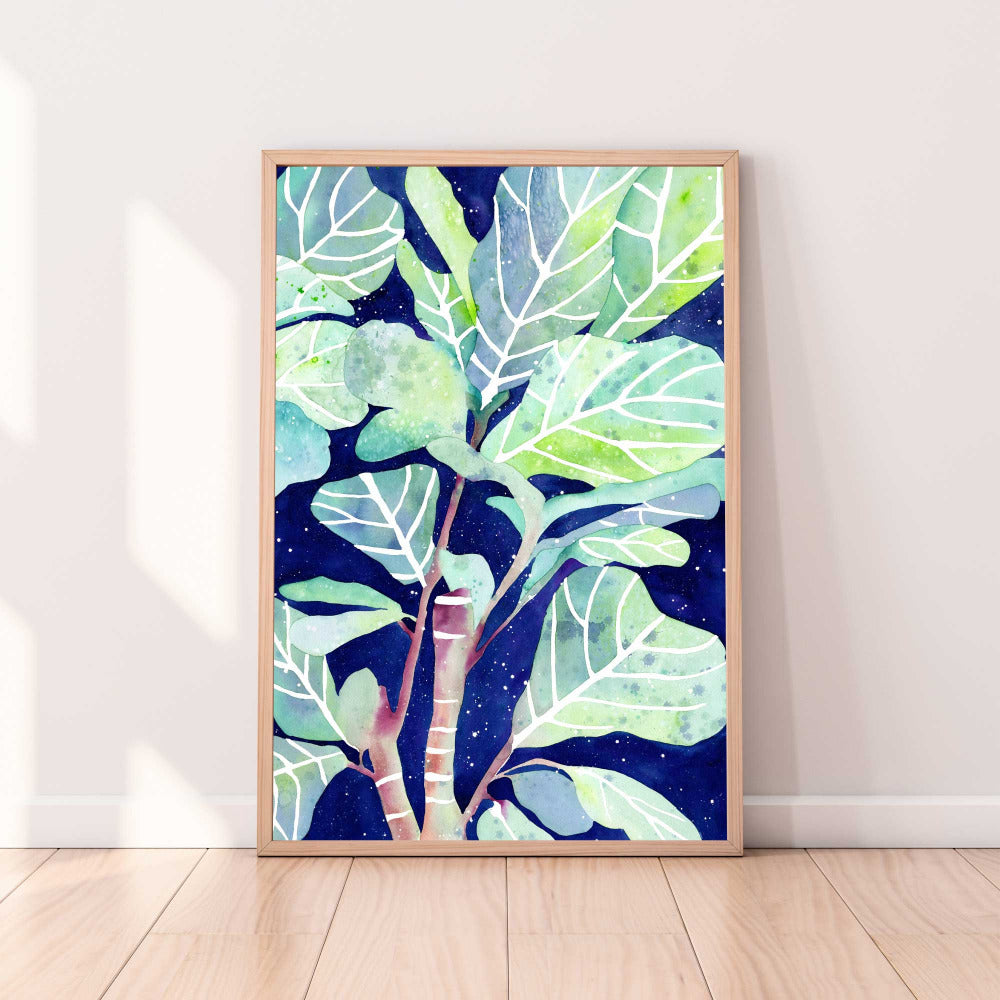The image features a vertical, rectangular, abstract watercolor painting propped up against a pale, off-white wall. The painting is framed in a thin, simplistic wooden frame that matches the light-colored, hardwood floor with visible grain patterns. The floor planks run vertically towards the wall. The artwork showcases a plant with two brownish stalks marked with white rings for bark segments. From these stalks, large, broad leaves extend, displaying a palette of pastel mottled greens, ranging from sea green to lime green, all highlighted by pronounced white veins. The background of the painting is a deep blue, dotted with small white specks, possibly evoking the imagery of a starry night sky.